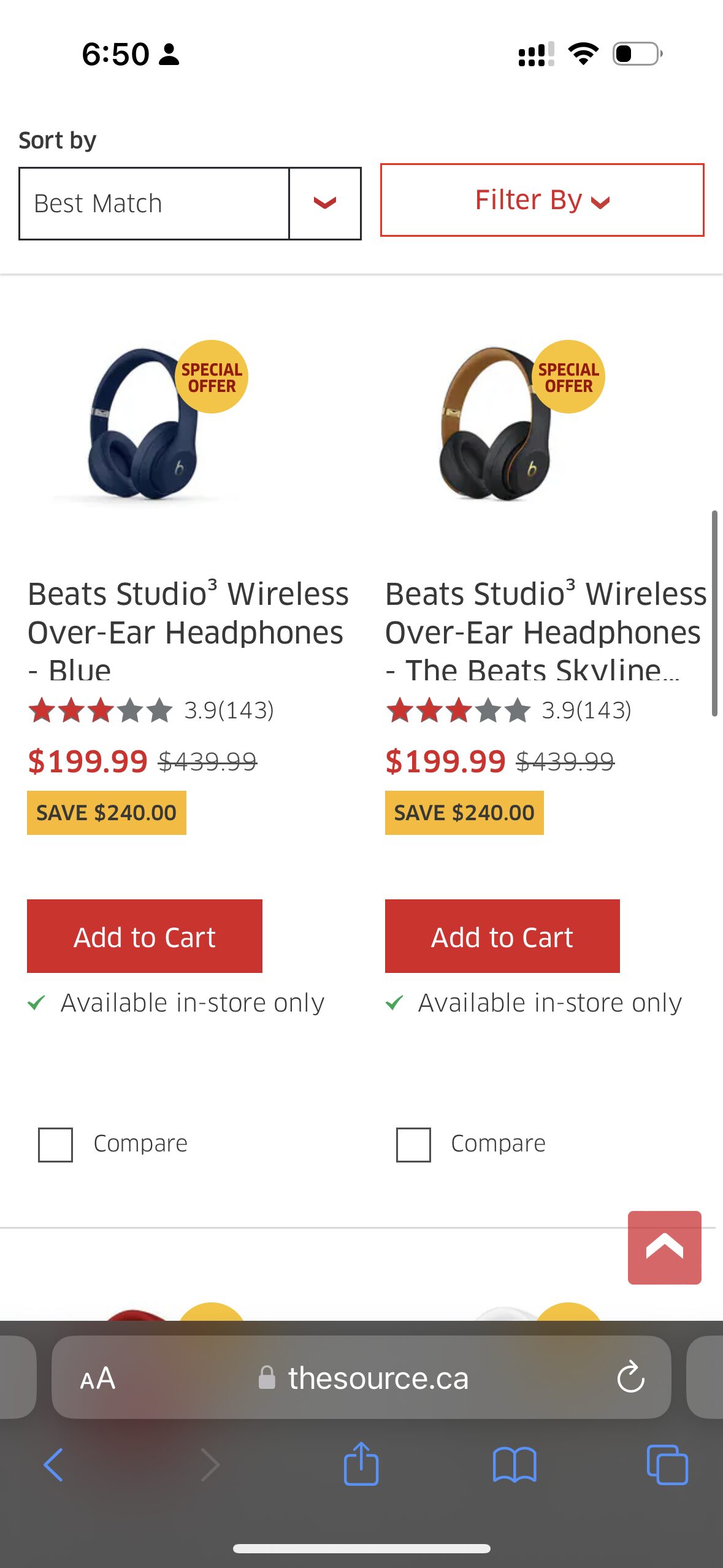This screenshot displays an unlabeled webpage, likely depicting a shopping platform, as seen from the various icons and elements present. The status bar at the top of the screen shows it is 6:50 (unspecified if AM or PM), along with a small person icon, three out of four signal bars, a Wi-Fi symbol, and a battery indicator showing approximately 25% remaining.

Below the status bar, the page presents two options for headphones, both labeled as "Special Offer." Users can sort by options such as "Best Match" or apply filters to refine their search.

The first product displayed is the Beats Studio Wireless Over-Ear Headphones in blue. It has a rating of 3.9 stars based on 143 reviews. The headphones are priced at $199.99, discounted from the original price of $439.99, offering a savings of $240. An "Add to Cart" option is available, although it notes the item is "Available In-Store Only." There is also a feature to compare this product with others on the list.

The second product listed is the Beats Studio Wireless Over-Ear Headphones, specifically the Beats Skyline edition. This product shares the same 3.9-star rating, albeit with 43 reviews. It is also priced at $199.99, with a discount from $439.99, saving shoppers $240. Similar to the first product, there is an "Add to Cart" option and a note specifying "Available In-Store Only." Users can also compare this item with others.

Overall, the webpage provides a concise overview of two discounted headphone options, assisting users in making an informed decision.